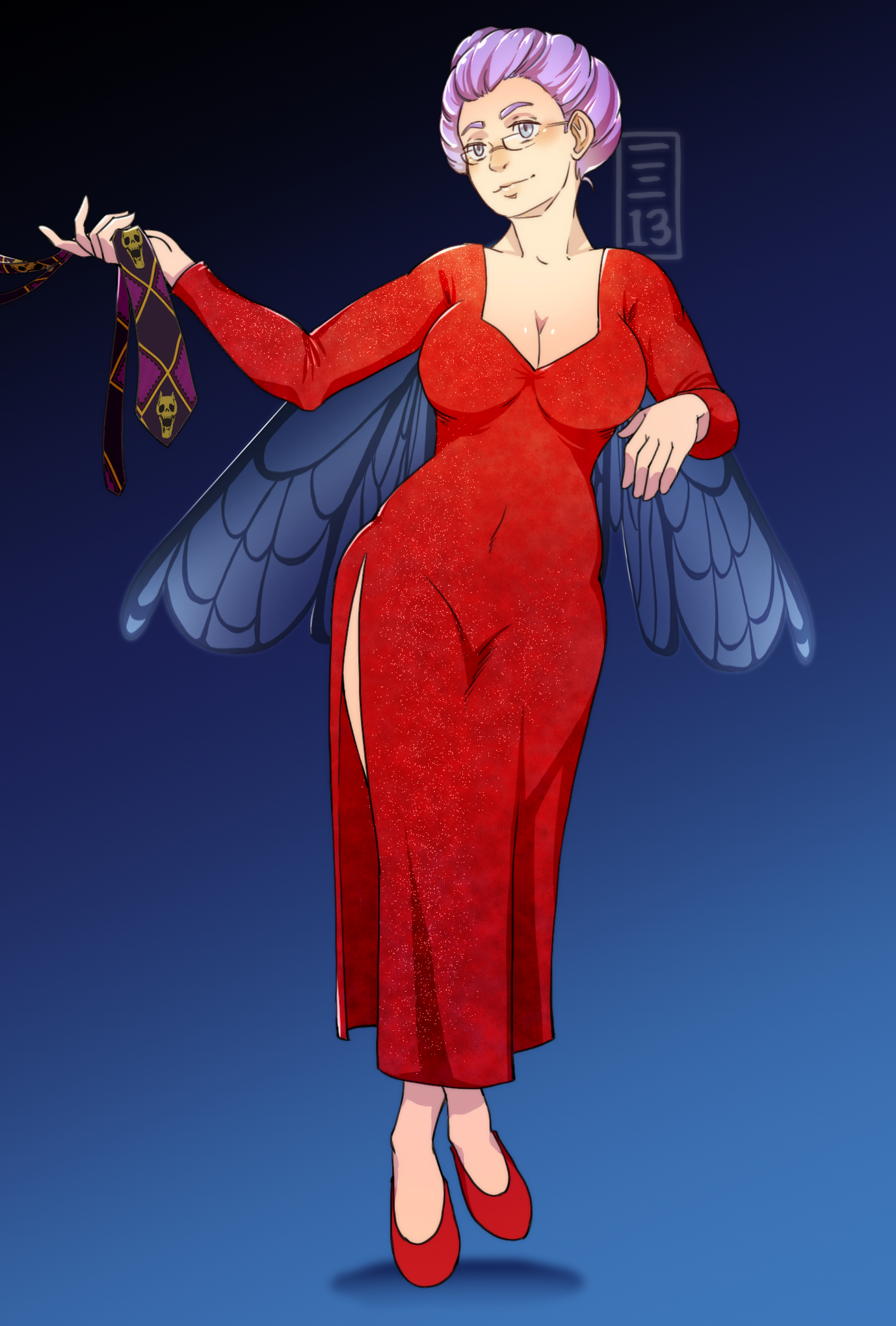The image showcases a digital artwork of an elderly woman with a youthful, shapely figure. She has light pink hair and her eyes are blue, partially obscured by glasses that rest low on her nose. She smiles gently while holding a tie adorned with yellow demonic figures and purple-black infinity symbols, along with a golden skull. The woman wears a revealing, form-fitting red dress with a high slit on one side, emphasizing her large chest. She stands on her tiptoes in red slippers, appearing to float above the ground with a shadow cast beneath her. Behind her, blue-toned insect-like wings are spread out. The background transitions from dark to a lighter blue towards the bottom, and in the upper left corner, there's a gray square with the number 13.